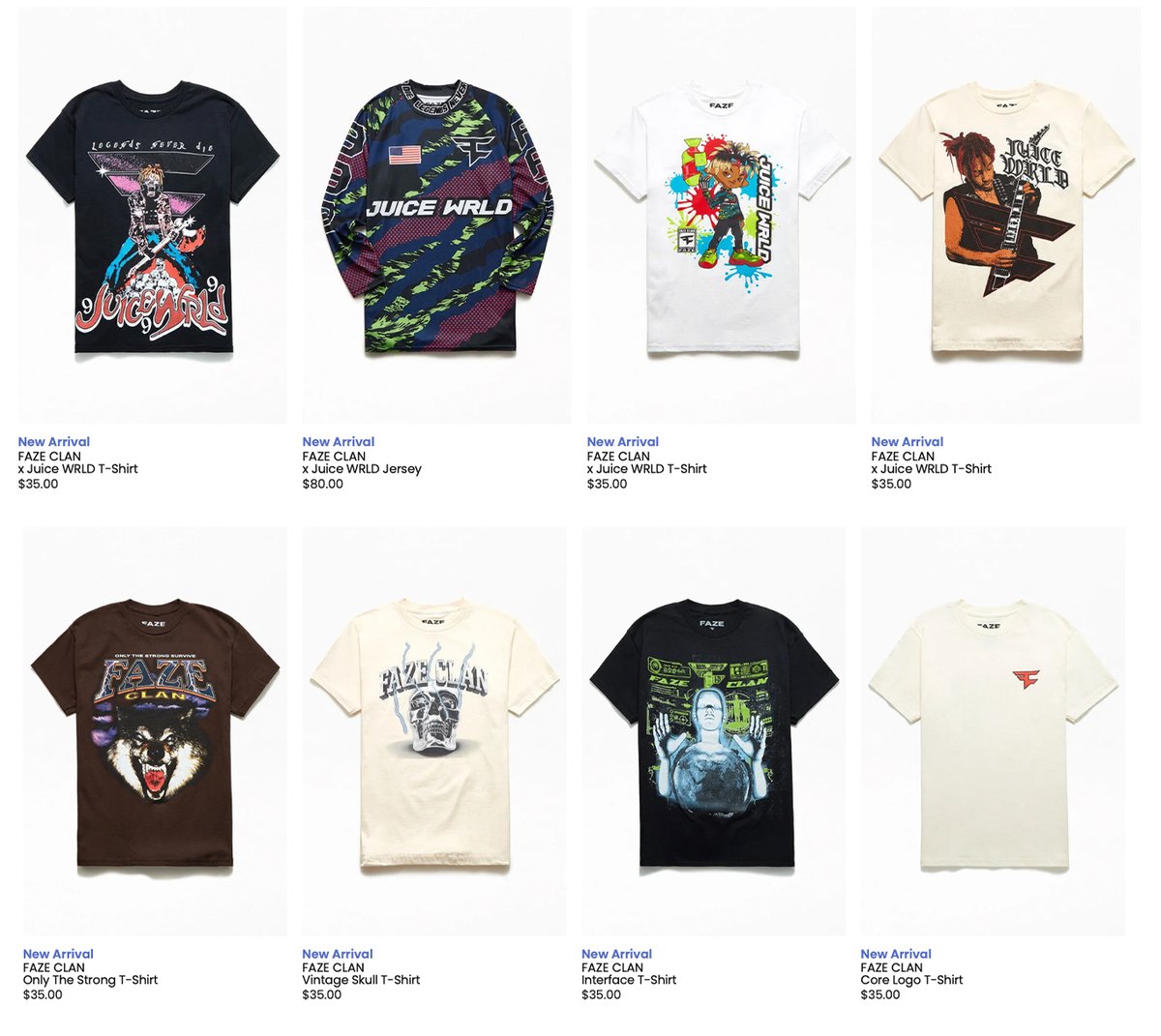Introducing the latest additions to the Faze Clan collection in collaboration with Juice WRLD and other unique designs:

1. **New Arrival Faze Clan X Juice World Skeleton T-Shirt:** A striking black t-shirt featuring a skeleton graphic and the words "Juicy". Priced at $35.

2. **New Arrival Faze Clan X Juice World Striped Long-Sleeve T-Shirt:** This eye-catching long-sleeve shirt combines green and purple stripes with "Juice World" lettering. Available for $80.

3. **New Arrival Faze Clan X Juice World Cartoon Character T-Shirt:** A white t-shirt adorned with a playful cartoon character and vibrant paint splatters. Priced at $35.

4. **New Arrival Faze Clan X Juice World Guitarist T-Shirt:** Featuring a graphic of a guy playing a guitar while wearing a vest, this black t-shirt is priced at $35.

5. **New Arrival Faze Clan "Only the Strong" Wolf T-Shirt:** This black t-shirt showcases a detailed graphic of a wolf's face. Available for $35.

6. **Faze Clan Vintage Skull T-Shirt:** A white t-shirt with "Faze Clan" lettering and a striking smoking skull design in the background. Priced at $35.

7. **Faze Clan Interface T-Shirt:** A black t-shirt featuring "Faze Clan" in green, accompanied by a blue orb-like object and a person with their hands up behind it. Available for $35.

8. **Faze Clan Core Logo T-Shirt:** A clean white t-shirt prominently featuring the signature red Faze Clan logo. Priced at $35.

Take your style to the next level with these fresh new arrivals from Faze Clan!